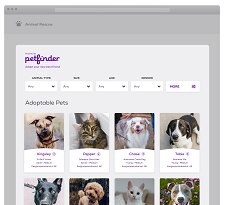This image, despite being somewhat blurry and difficult to make out, shows a website layout with several distinct sections. At the top, there is a URL box, followed by a dark gray band featuring a paw print logo with the text "Animal Something." Beneath this, a lighter gray section displays the name "Pet Finder" in dark purple cursive writing, accompanied by an illegible slogan above and below. The image also includes five drop-down menus, each labeled to guide user interactions, with the one on the far right marked with the word "More" in purple text. Directly below this, in black text, it says "Adoptable Pets," and showcases eight images of cats and dogs arranged in two rows of four.